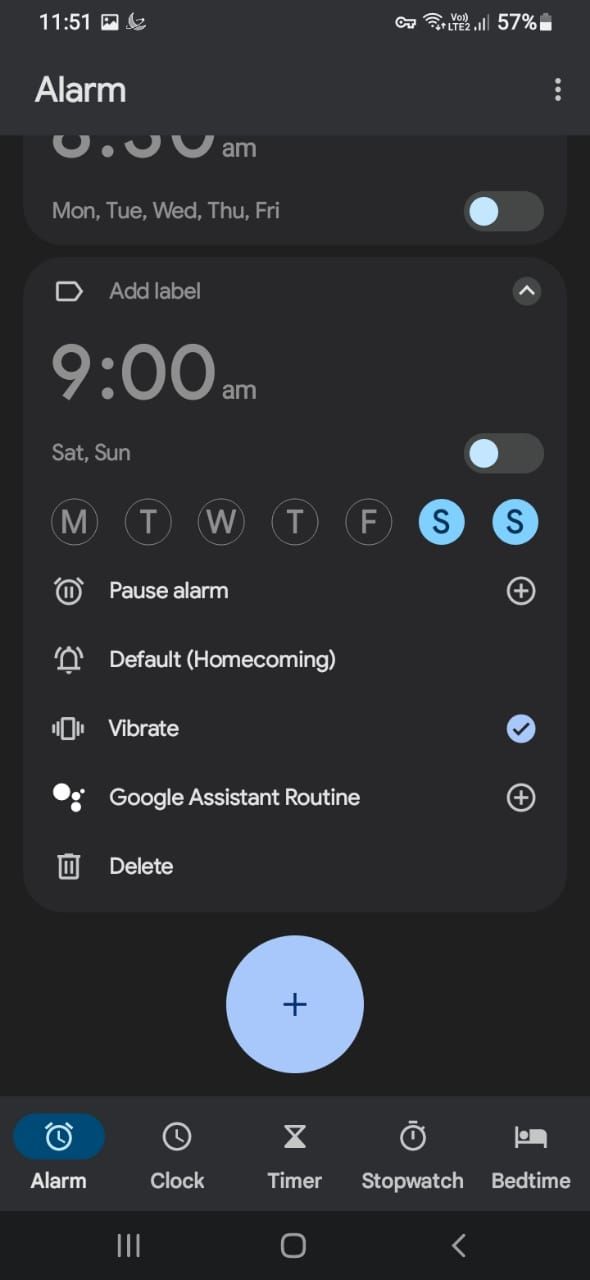The image displays a sophisticated user interface of a digital alarm application. At the top, the screen indicates the current time as "11:51", with a key symbol labeled "415". The battery indicator is visible but suggests a low battery warning.

The center of the screen has various alarm settings, with a focus on days of the week. A notable alarm is set for "Friday," but it appears this setting isn’t toggled on. There are additional unverified alarms for "Saturday" and "Sunday."

The interface features an array of icons including:
- A circle with a plus sign outline on a gray background, representing the option to add new alarms.
- A bell icon indicating notifications.
- A vibrating circle with a checkmark signifying completed or acknowledged alarms.
- A "Google Assistant Routine" icon for setting up automated routines.
- A trash can icon for deleting alarms or settings.

At the bottom of the screen, there is a light blue circle featuring a plus sign, designated for creating new alarms or reminders. 

The application provides several functions:
- An oval clock icon indicating the current active alarm.
- Navigation buttons for "Clock", "Timer", "Stopwatch", and "Bedtime" features.
- A hamburger menu for additional settings and options.
- A sideways arrow within a square icon, possibly for navigating to previous screens.
- A faint gray bar at the bottom framing the interface, likely for device navigation.

Overall, the interface is predominantly gray with light blue highlights, providing a modern and functional design focused on time management and alarm settings.